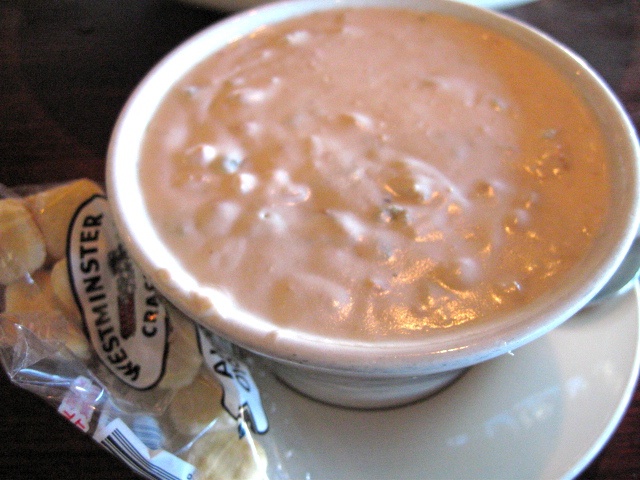The image depicts a bowl of thick, creamy soup, likely clam chowder, given its lumpy texture and whitish color, set in a white bowl on a matching white plate. Both the bowl and the plate are placed on a dark tabletop, creating a contrasting backdrop. To the left of the bowl, there is a clear plastic package of soup crackers, partially displaying the brand name "Westminster" and the letters "CRA" from the word "crackers". The soup appears to be lukewarm and has a slightly pale orange hue. A spoon’s handle is visible, protruding from the side of the bowl, adding to the setting’s ambiance, which hints at a possible restaurant environment.